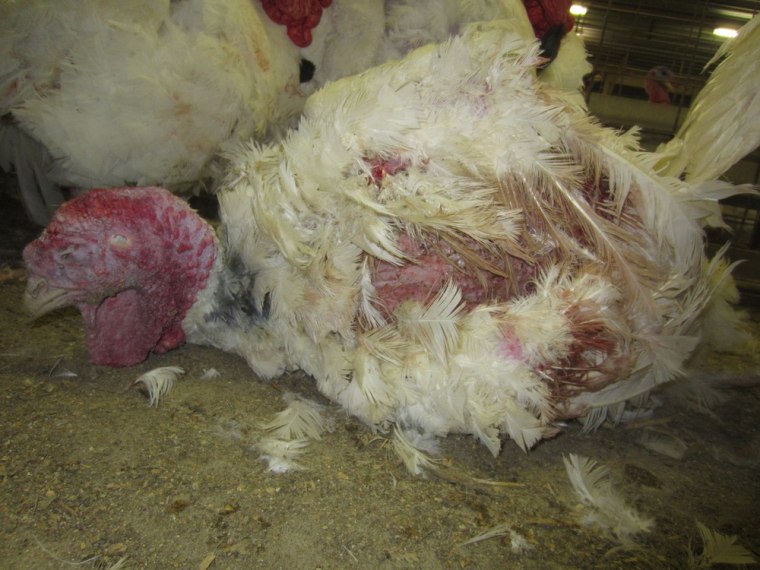In this detailed photograph, we observe an injured young turkey within a large-scale turkey farming operation. The animal, small in size and lying on a dirt floor mixed with grit and soil, presents a disturbing picture with its missing and broken white feathers. The pink and red skin beneath the few remaining feathers, including the turkey’s neck and head, suggests damage and possible injury. Its light-colored beak and almost closed eyes further emphasize its poor condition. Scattered feathers around the turkey add to the scene of distress. In the background, more white turkeys are visible, with a view of the farming environment marked by low walls, bars, metal grids, and a roof, indicating the enclosure of a crowded pen. The poor turkey is surrounded by other birds in similarly close and confined quarters.